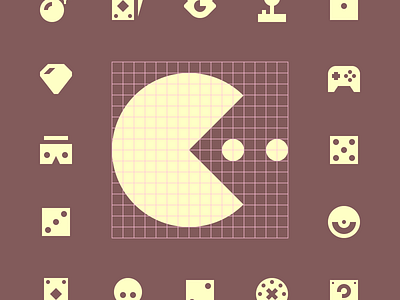In the center of the image is a square art panel featuring a light tan Pac-Man character with its mouth open, seemingly gobbling up two light tan cookies. The Pac-Man character is set against a background that oscillates between a dark tan and a purplish haze. Overlaying the Pac-Man scene is a light pink grid, adding an extra layer of texture to the composition.

Surrounding this central panel is a border filled with various gaming-related symbols and geometric shapes, organized in a square pattern. These include several dice showing different numbers like one, three, and five, a square with a question mark, and shapes reminiscent of card suits and VR goggles. Additionally, there are symbols familiar to vintage computer games, such as different types of joysticks and a circle with an X and surrounding dots. Altogether, the image blends a nostalgic gaming aesthetic with an organized yet seemingly random assortment of iconic symbols, evoking a retro, game-inspired art piece.